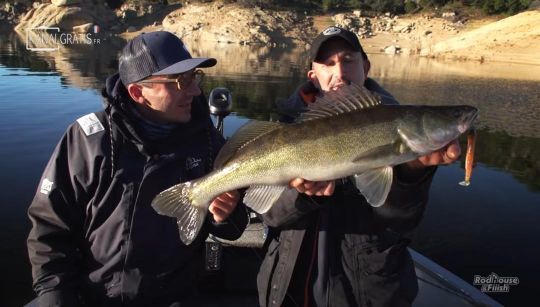In this detailed photograph, two men are out fishing on what appears to be a lake during the late afternoon, evidenced by the deep shadows and dark colors with only some patches of illuminated ground. Both men, who are in a small boat equipped with a trolling motor, serve as the focal point. They are each dressed in black waterproof winter jackets and dark navy blue or black baseball caps. The man on the right, sporting a mustache, is proudly displaying a sizeable fish that is likely around 20 inches long, characterized by its greenish-silver hue and darker upper body. The fish has a large lure dangling from its mouth. Both men are facing the viewer, although the man on the left, wearing glasses, is looking intently at his companion to the right. The backdrop features dark-colored, reflective water and a shoreline of brown, rocky terrain sporadically dotted with trees or bushes. Notably, a logo in the bottom right corner reads "Rod House Fish," suggesting the image may be associated with a television or internet fishing show.